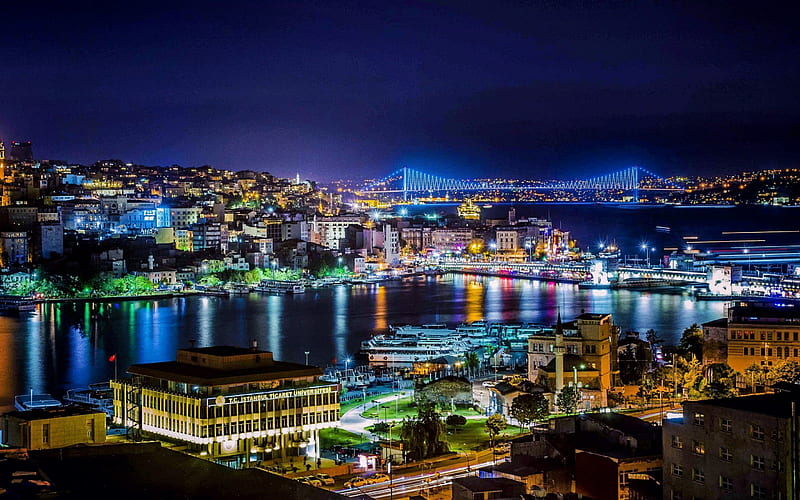This stunning nighttime image captures a vibrant cityscape featuring a city built around water. A magnificent blue-lit bridge spans the waterway in the distance, while another illuminated bridge crosses a nearby canal or river. The buildings are bathed in a golden glow, interspersed with trees adorned in green lights and some structures lit up in pink. The scene is bustling with activity and dense with residential lights climbing up the hills on both sides. In the foreground, a set of tugboats is visible alongside a prominent larger building and two other noticeable structures, all contributing to the lively and picturesque atmosphere.